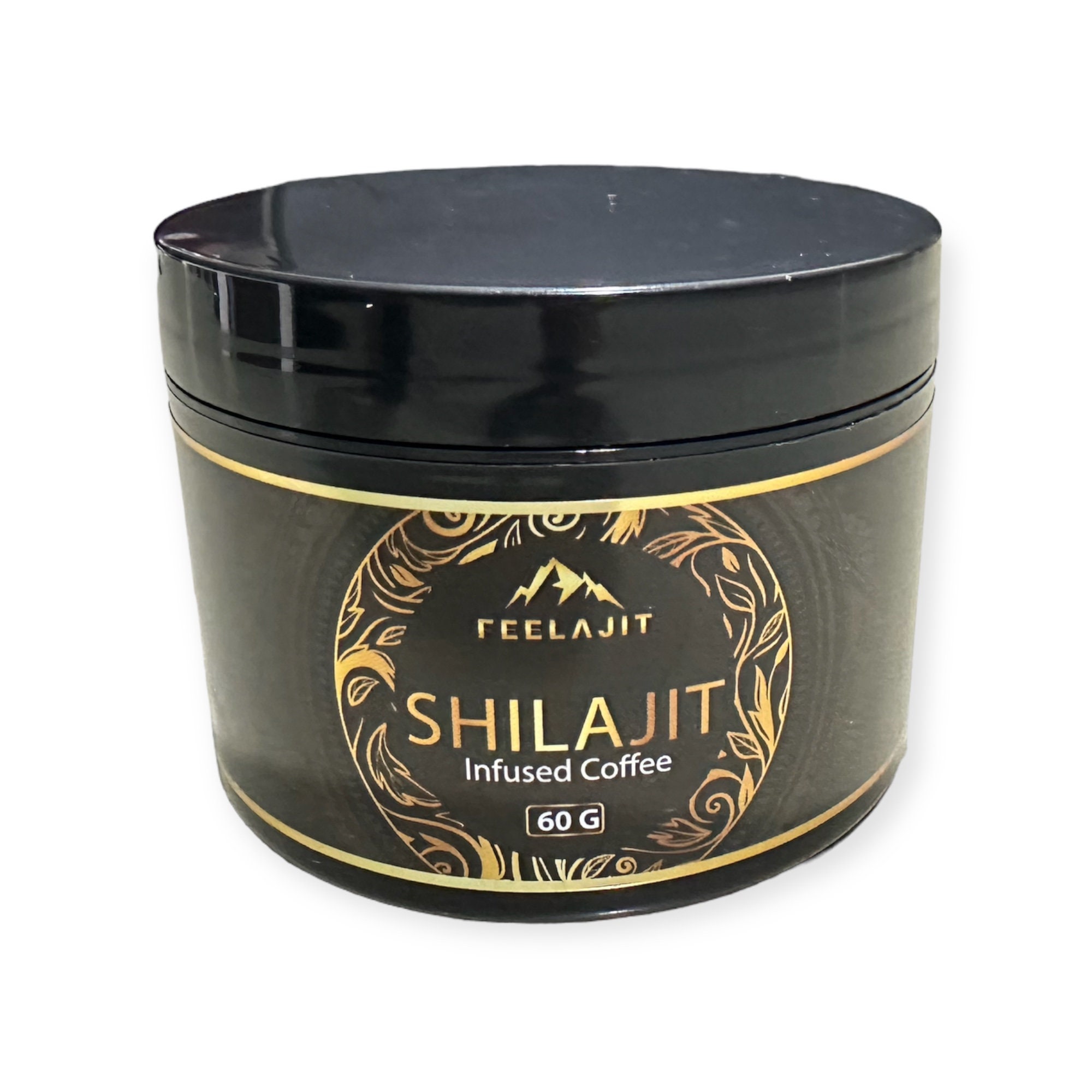This advertising image features a sleek, black cylindrical container with a screw-on lid, set against a stark white background. The container, made of heavy plastic, shimmers and reflects its surroundings. Dominating the front of the container is a stylish gold label enveloped by a decorative pattern of leaves. The label showcases a circular logo with an illustration of a mountain at the top. Below the mountain, in elegant gold lettering, is the brand name "F-E-E-L-A-J-I-T," followed by the product name "S-H-I-L-A-J-I-T" in larger gold letters. Beneath this, "Infused Coffee" is printed in white, and at the very bottom, the weight "60G" is indicated.